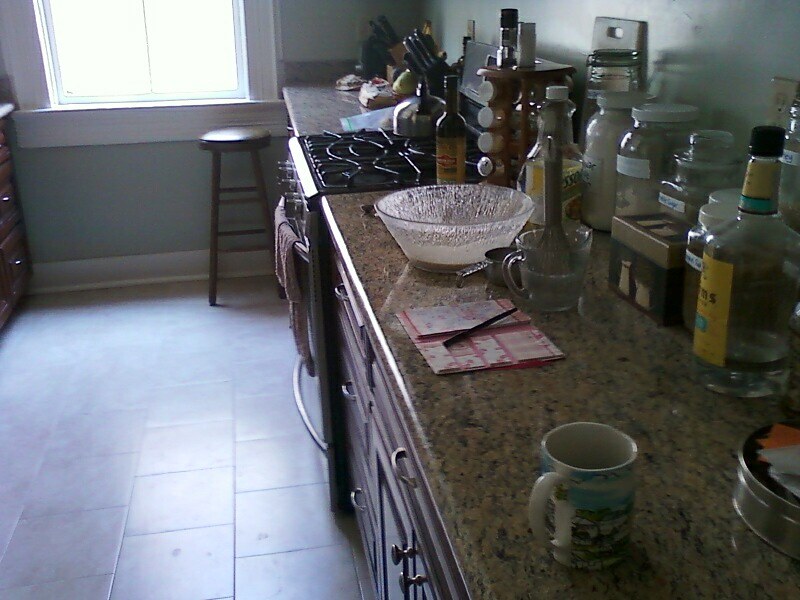This photograph captures a cozy and eclectic kitchen space. At the forefront is a long countertop, possibly made of granite or faux granite, featuring a rich brown and black mottled design. In contrast, the countertop towards the back of the room appears to be a laminate surface with a retro mix of white, pink, and blue hues. The kitchen extends towards the far end where a window brightens the room. Positioned near this window is a stool, suggesting a cozy spot for a quick bite or a leisurely coffee, facing a smaller countertop that could serve as a breakfast bar.

Adjacent to this bar area stands a stovetop with an oven beneath it, framed by another section of counter devoted presumably to food preparation. Adding to the kitchen's character is a wooden, rotating spice rack filled with assorted spices. The space is dotted with personal touches and practical kitchen items: several bottles of alcohol, large mason jars containing white and brown sugar, a muddler, a measuring cup, and a large crystal bowl. A mug, some napkins, a pen, and stationery add a hint of everyday living to this vibrant culinary hub.